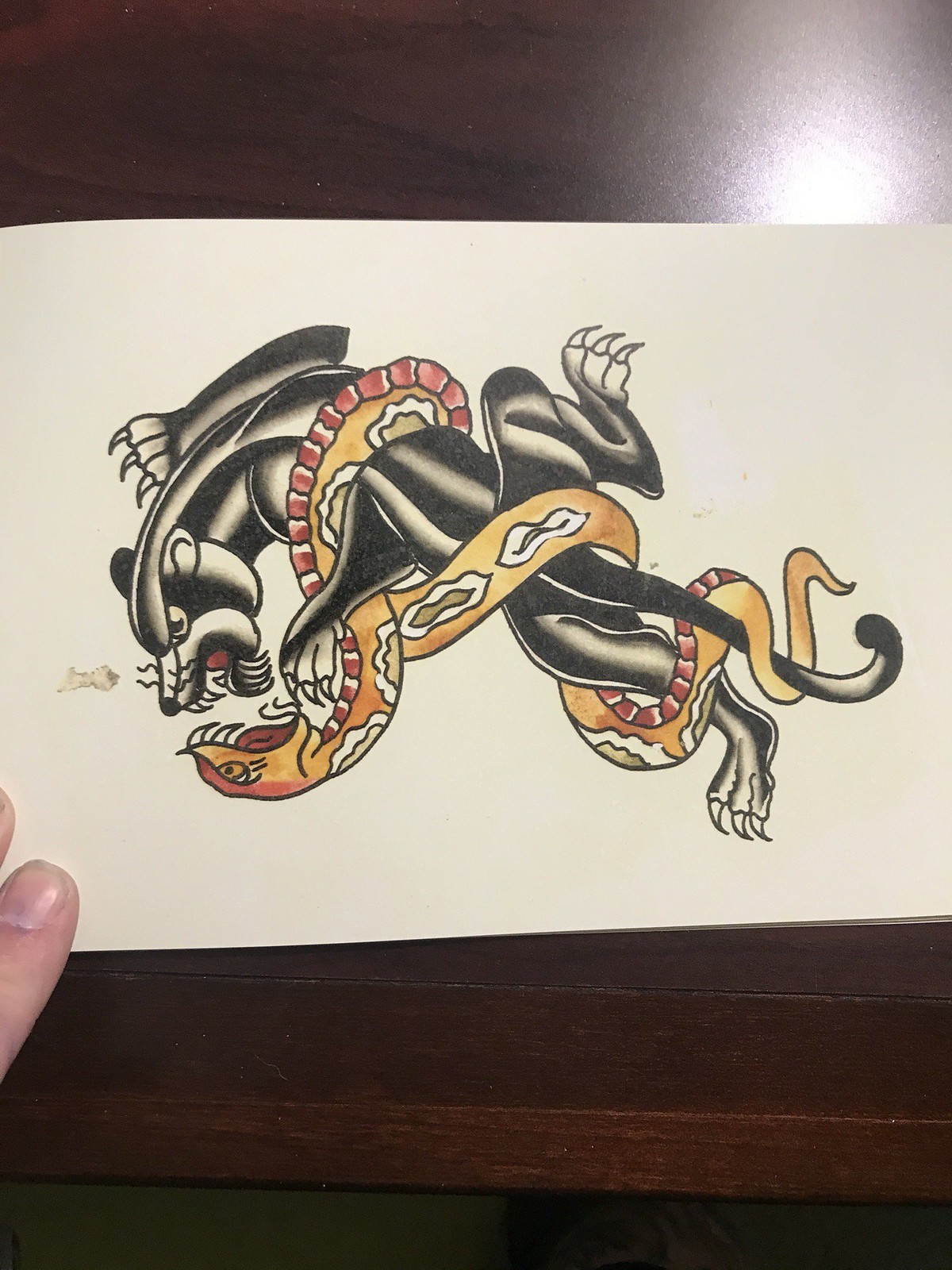In the image, there is a strip of paper lying on a flat surface, partially covered by a hand positioned to the left side. The paper features an intricate drawing of a creature that resembles either a black cat or a badger, characterized by its black and white fur. The creature's claws are distinctly white. Encircling this creature is a large, formidable snake. The snake’s body is adorned with a striking pattern: it has a vivid red belly, bordered by white edges. Within these white patterns, a brown coloration adds further detail. The snake's head is depicted in an aggressive stance, with its mouth wide open, revealing a red interior. The scene captures a sense of tension and complexity, blending natural elements into a visually compelling composition.